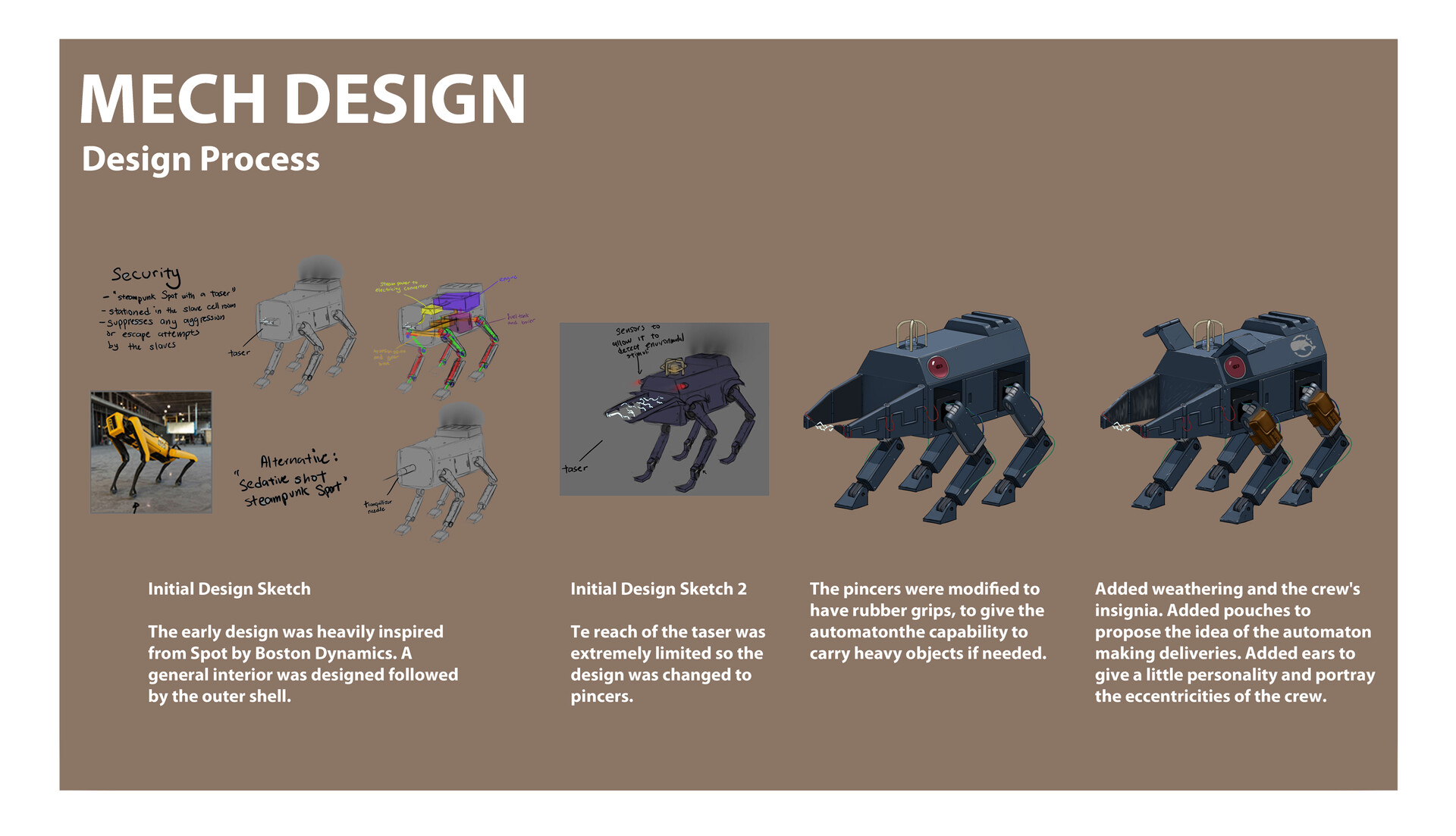Here is a single, detailed caption combining the information from all three descriptions:

---

**Mech Design Design Process**

The image portrays a comprehensive view of the design evolution of a large, yellow mechanical grasshopper-like robot, set against a taupey brown background. In the top left corner, the title "Mech Design Design Process" is written in white text. On the left side of the image, "Security" is written in black text. 

The image sequence begins with sketches of the robot, detailing the different stages of its design. The initial design sketch, labeled as "initial design sketch," reflects early inspirations from Spot by Boston Dynamics. The first illustration focuses on the general interior structure, followed by the outer shell. The image shows the initial concept altered to modify design features, such as the reach of a taser mechanism being replaced with pincers due to limited reach.

Moving to more advanced stages, the next illustration provides a 3D rendering of the robot, where the pincers are modified to have rubber grips, enabling the robot to carry heavy objects. Throughout the design, additional attributes like weathering, crew's insignia, and pouches are added, suggesting the robot's capacity for making deliveries. The final touches include added ears to give the robot a characteristic personality, reflecting the eccentricities of its creators.

An inset image showcases a detailed finish of the robot, represented as a black and yellow machine, placed on what appears to be asphalt. Surrounding this, there are multiple iterations of the robot in various stages: gray prototype sketches, colored renderings showing internal components, and finalized models given realistic textures and markings.

Overall, the image not only documents the step-by-step development from concept to final product but also highlights the practical and aesthetic modifications made throughout the design process.